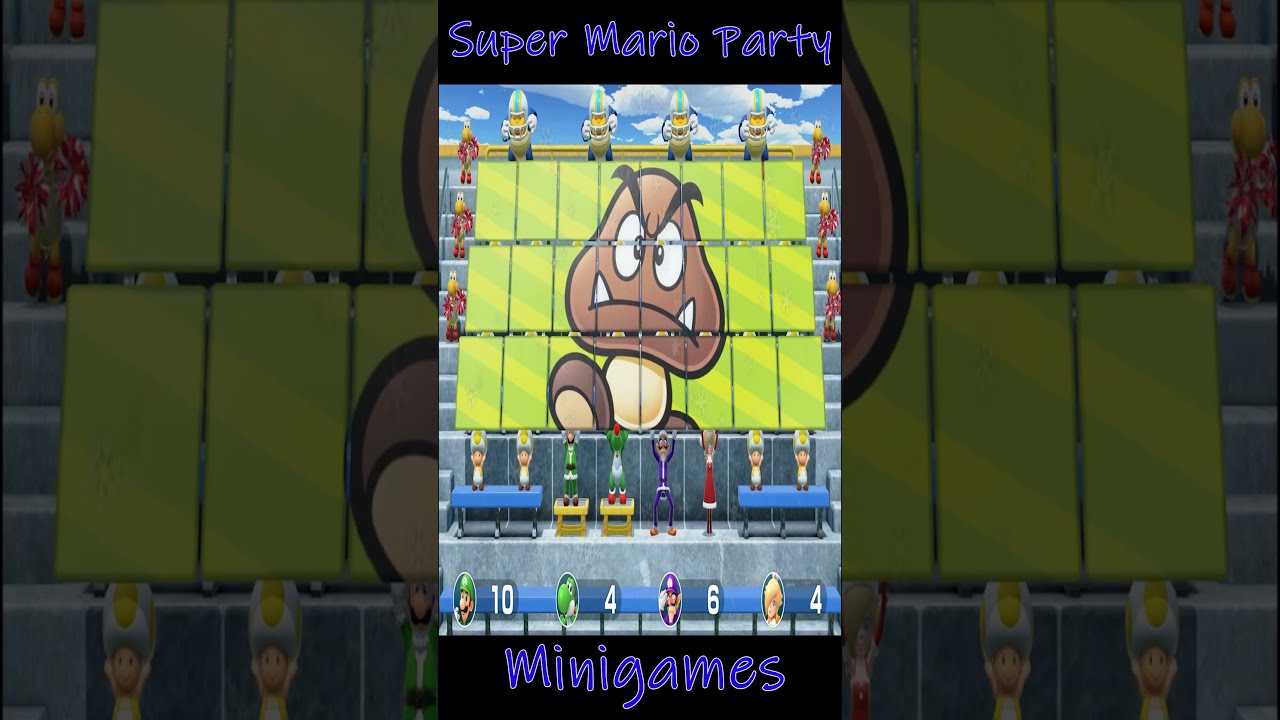This color image appears to be a screenshot from the video game "Super Mario Party," taken in portrait orientation. At the top and bottom of the screen, against a black background, blue text displays "Super Mario Party" and "mini games," respectively. The central portion of the image features a segmented, yellowish playing field with a prominent, brown cartoon character that resembles a snakehead or dinosaur. This character has two upward-pointing white teeth and dark, menacing eyebrows. Surrounding this central figure are various characters from the Mario universe, positioned at the top, sides, and bottom of the field. Notable characters include Mario and Luigi at the bottom, accompanied by white numbers 10, 4, 6, and 4, indicating different scores. The background features a sky with blue skies and white clouds, providing a vibrant and animated setting.